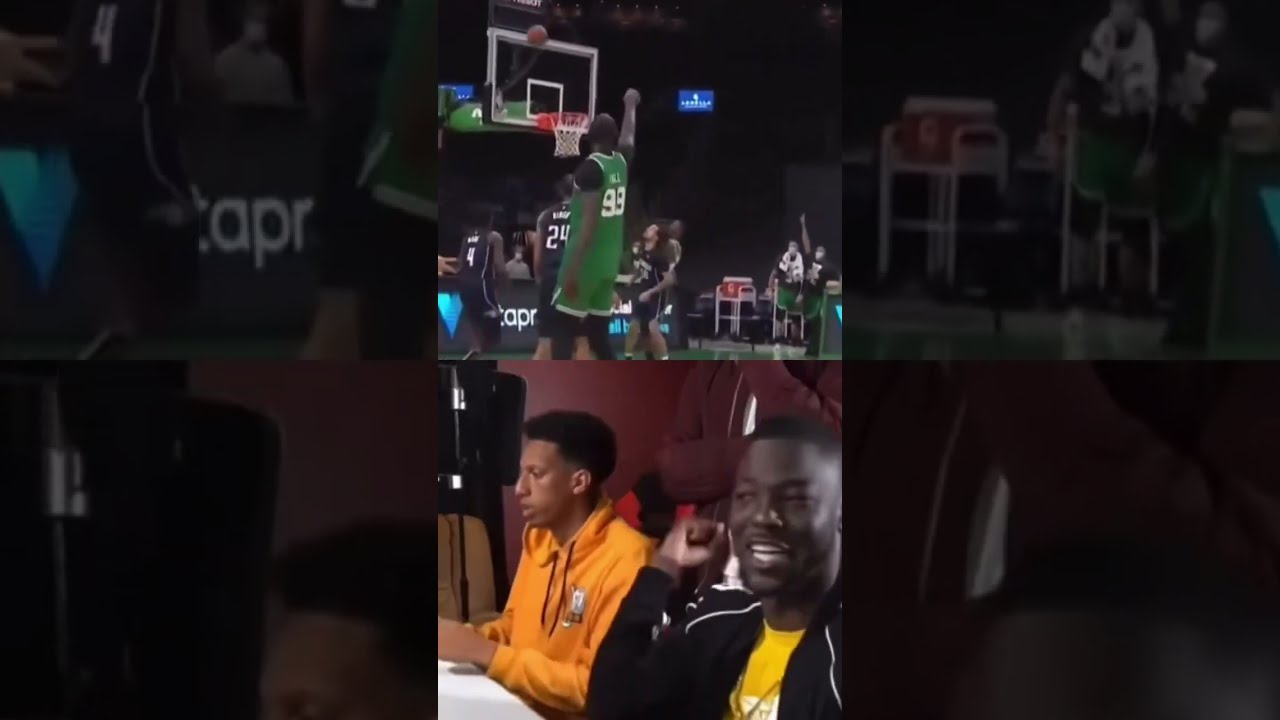The image is a combination of two stacked color photographs. The top picture depicts a dynamic moment from a Boston Celtics basketball game, capturing a player in a green jersey, number 93, who has just released a shot towards the clear backboard and red hoop. Other players in black jerseys, including one with the number 24, are visible around him. This capture includes a translucent barricade on the court and a partially-viewed crowd in the background, adding to the lively atmosphere of the game. 

Below, the bottom picture shows two African-American men seated at a table covered with a white cloth, seemingly in a recording studio or similar setting with red walls. The man on the left, wearing a black jacket over a yellow shirt, is smiling, while the man on the right dons an orange hoodie. Additional details include speakers and another individual in the background, contributing to the impression of a commentary or reaction setup. This combination suggests that the bottom image is likely a reaction or meme related to the basketball game depicted above, possibly implying a humorous or critical response to a particular play in the game.